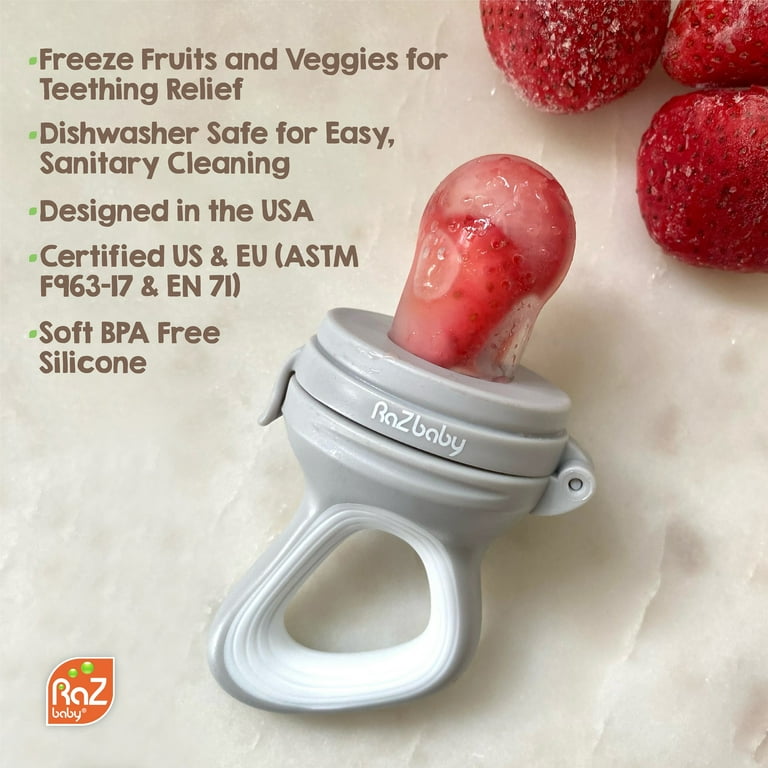This advertisement showcases a unique baby pacifier designed for teething relief. The gray and white pacifier features a hinged clip that allows you to insert frozen fruits or vegetables, such as a strawberry, into the white silicone nipple. In the upper left corner, there are bullet points with green dots written in brown text highlighting its key benefits: "Freeze fruits and veggies for teething relief," "Dishwasher safe for easy, sanitary cleaning," and "Designed in the USA, certified US and EU ASTM F 963." Additional details include "Soft BPA free silicone" and the RAZ baby logo at the bottom. The background appears icy or cold, emphasizing the pacifier's cooling relief for teething babies.